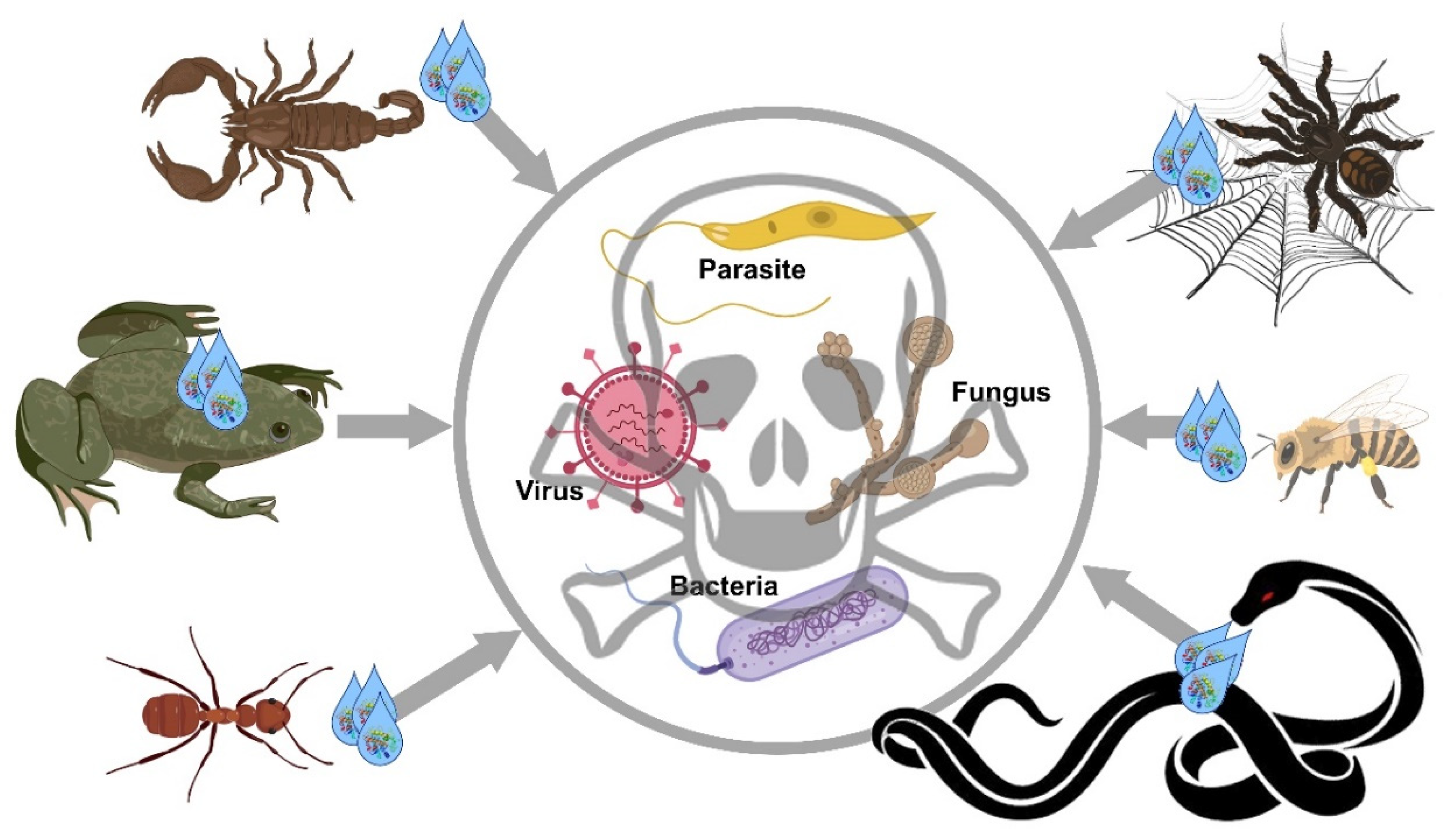This infographic illustrates the transmission of various pathogens through small animals and insects, depicted in a central circular diagram. At the heart of the image is a gray-lined circle featuring a skull and crossbones, symbolizing danger or toxicity. Inside this central circle are detailed representations of different pathogens: a yellow worm labeled "parasite" at the top, an image of a virus on the left, a fungus on the right, and bacteria at the bottom. 

Surrounding this central area are six animals, each associated with droplets or water sources, and indicated with arrows pointing toward the middle, signifying their role in transmitting these pathogens. On the left side, there is a scorpion at the top, a frog in the middle, and an ant at the bottom. On the right side, a spider is at the top, followed by a bee in the middle, and a snake at the bottom. This infographic effectively showcases how these animals and insects are vectors for spreading parasites, viruses, fungi, and bacteria.